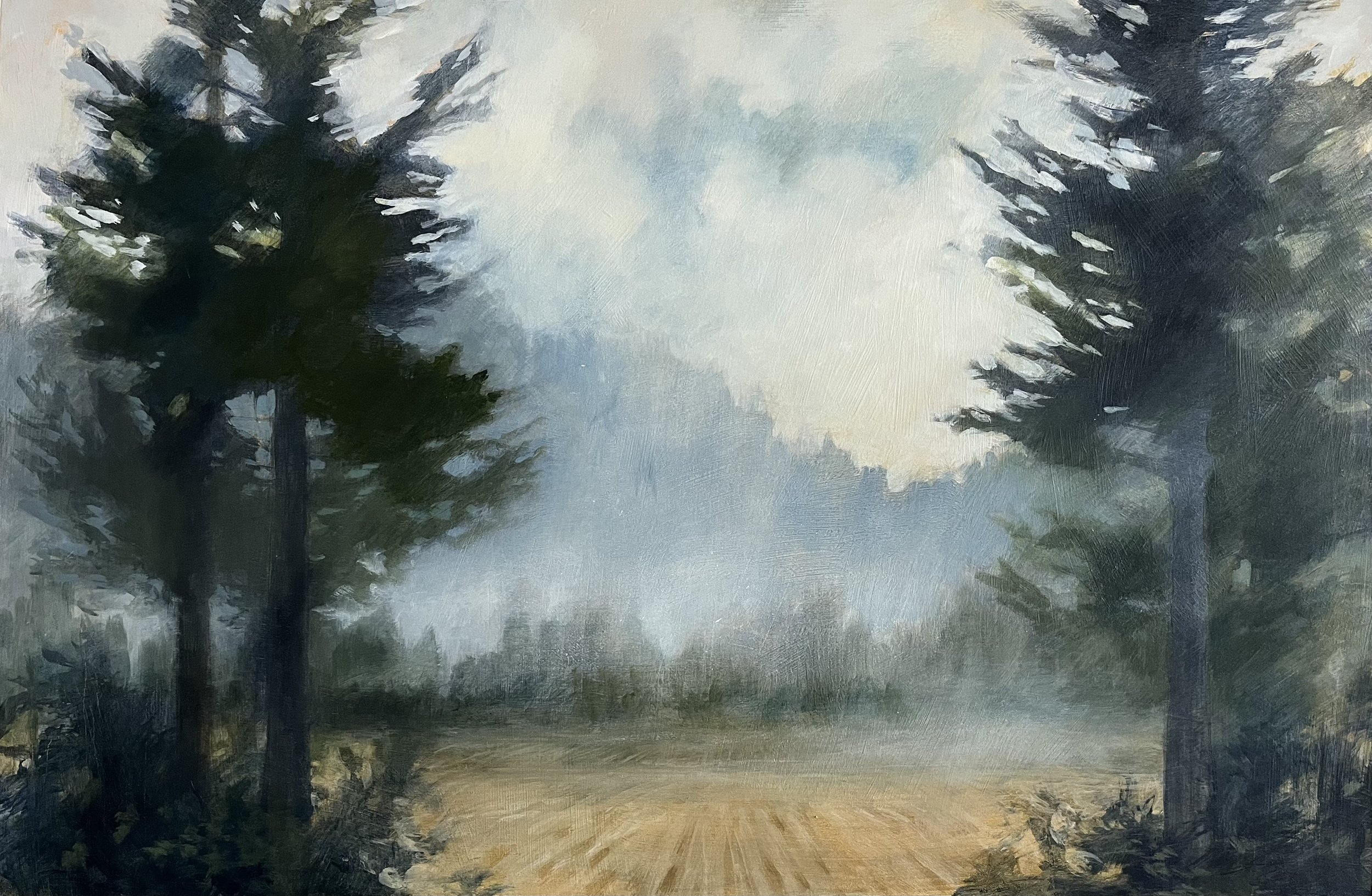The painting is an impressionistic depiction of a forest clearing, characterized by loose and varied brush strokes that create a somewhat blurry and abstract effect. Dominating the foreground are two large trees on the left and a single tree on the right, framing the scene and giving a sense of depth. Between these trees lies a dirt path that meanders from left to right through the center of the clearing. The middle ground features an open, greyish field that blends softly into surrounding trees and bushes. In the far distance, vague representations of mountains can be seen, adding to the painting's depth. The sky overhead is filled with white clouds, contributing to a slightly misty atmosphere. The overall composition is not sharply defined but remains clear enough to discern the elements within the scene, evoking the sensation of viewing through a hazy lens or the bottom of a glass. The use of oil paint and the impassioned brushwork give the painting a rich texture and a freeform, almost abstract quality.